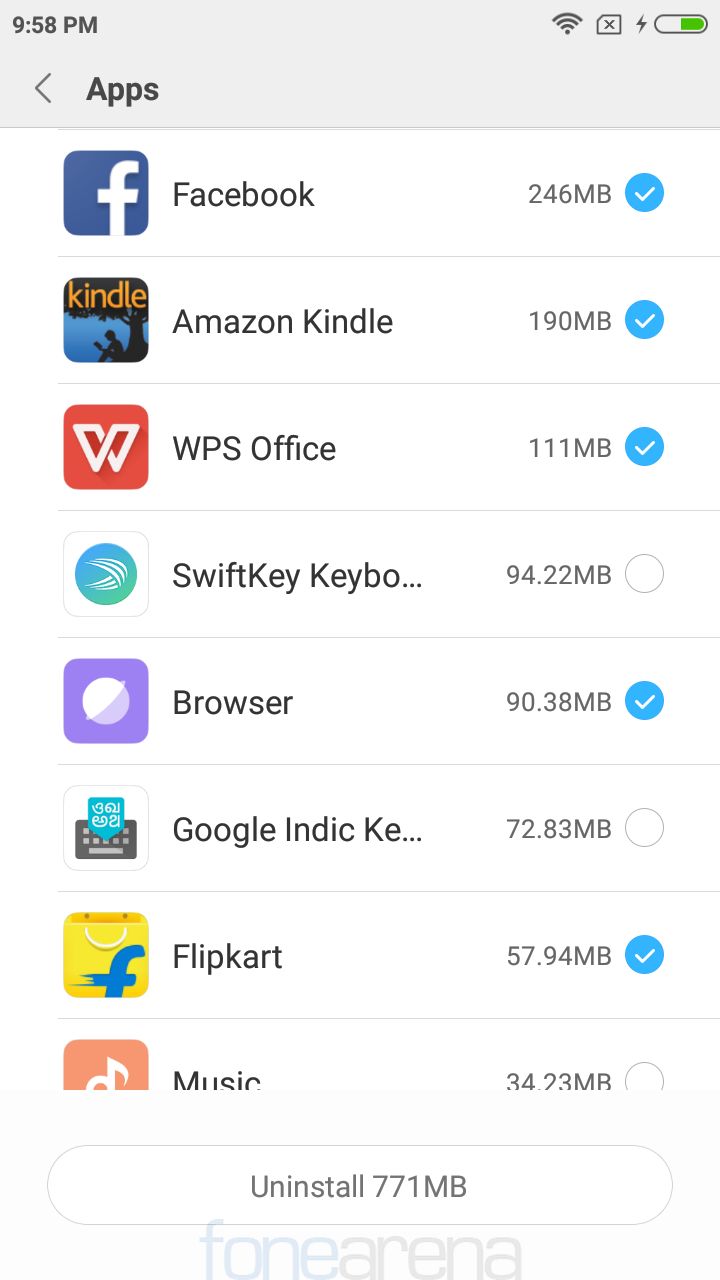**Detailed Caption:**

This image is a screenshot of a mobile phone application. At the top left of the screen, the light gray header displays the time "9:58 p.m." in dark gray font. On the top right, four icons are present. The rightmost icon is a pill shape, half-filled with a green bar on the right side, indicating some form of status or progress.

Below the header, toward the left, there is a grey arrow pointing left, followed by the word "Apps" in black text. Directly beneath this text, a thin medium gray shadow marks the boundary between the header and the main body of the application.

The body of the application has a clean white background and showcases a list of app icons along with relevant information. Each entry in this list features a name written in black text, followed by some negative space, and then a number indicating the app size in medium gray text accompanied by "MB". On the far right of each list item, there is a circular icon with varying styles.

Each item in the list is separated by thin light gray lines that extend across the screen from the left edge of each icon to the right side of the page.

The list of apps with their respective sizes (from top to bottom):
- Facebook: 246 megabytes
- Amazon: 190 megabytes
- Kindle: 111 megabytes
- WPS Office: 94.22 megabytes
- SwiftKey: 90.38 megabytes
- Keyboat: 72.83 megabytes
- Browser: 57.93 megabytes
- Google: 34.23 megabytes
- Indic: KE (text partially obscured)
- Flipkart: (size not specified)
- Music: (size not specified)

Overall, the interface is clean and well-organized, clearly displaying important information regarding the app usage in a user-friendly manner.